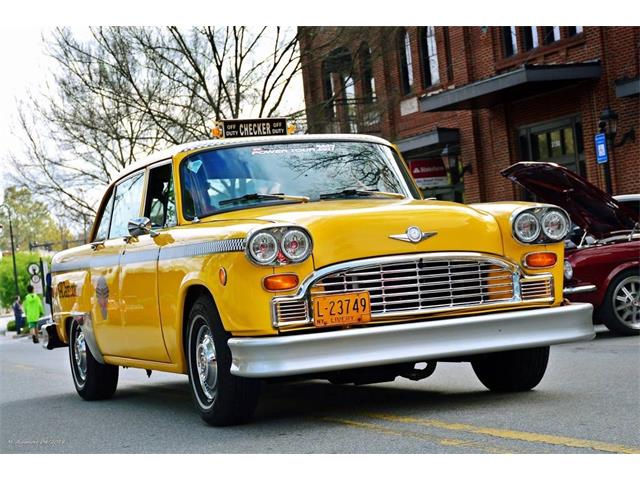This is a detailed photograph of a vintage yellow Checker taxi cab driving down a street, with its tires encroaching over the double yellow line in the middle of the road. The bright yellow cab has a distinctive boxy shape, a striking large chrome grille spanning the front, and four circular headlights—two on either side, with two round lights in each headlight cluster, and orange rectangular lights beneath them. The taxi has a black sign on its roof with the word "CHECKER" in white, flanked by the words "OFF DUTY" on both sides. The front license plate reads "L-23749." The car's tires are adorned with a white ring around them. Reflecting the sky and trees, the windshield obscures the interior, making the driver and potential passengers indiscernible. To the right of the frame, a red car with its hood open is parked outside a brick building next to a barren tree. Above the cab, leafless trees are visible against the sky, and in the background, a man in a neon green hoodie walks down the street.